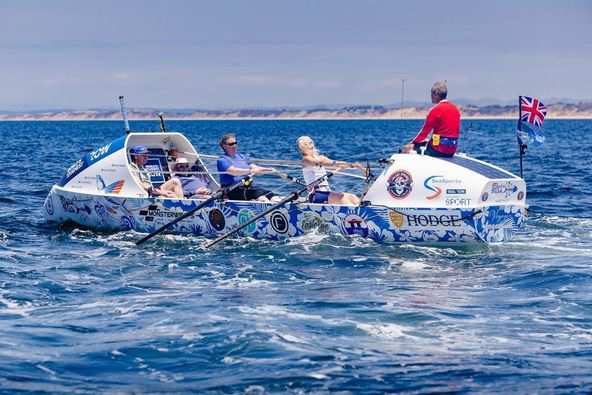This vibrant photograph captures a colorful, design-adorned rowing boat cutting through the blue, slightly wavy ocean under a mostly clear blue sky with minimal white clouds. The boat prominently features advertisements and logos, including the text "Hodge," and is adorned with both the USA and United Kingdom flags at its ends. Onboard, two women are actively rowing from the center of the boat while two men behind them, and another man up front, observe, potentially coordinating the effort. The boat, heading left to right in the frame, is surrounded by a scenic backdrop that includes a bit of white and gray coastline and faint mountains in the distance. The overall scene suggests an outdoor, daytime maritime activity possibly observed from a nearby boat at eye level.